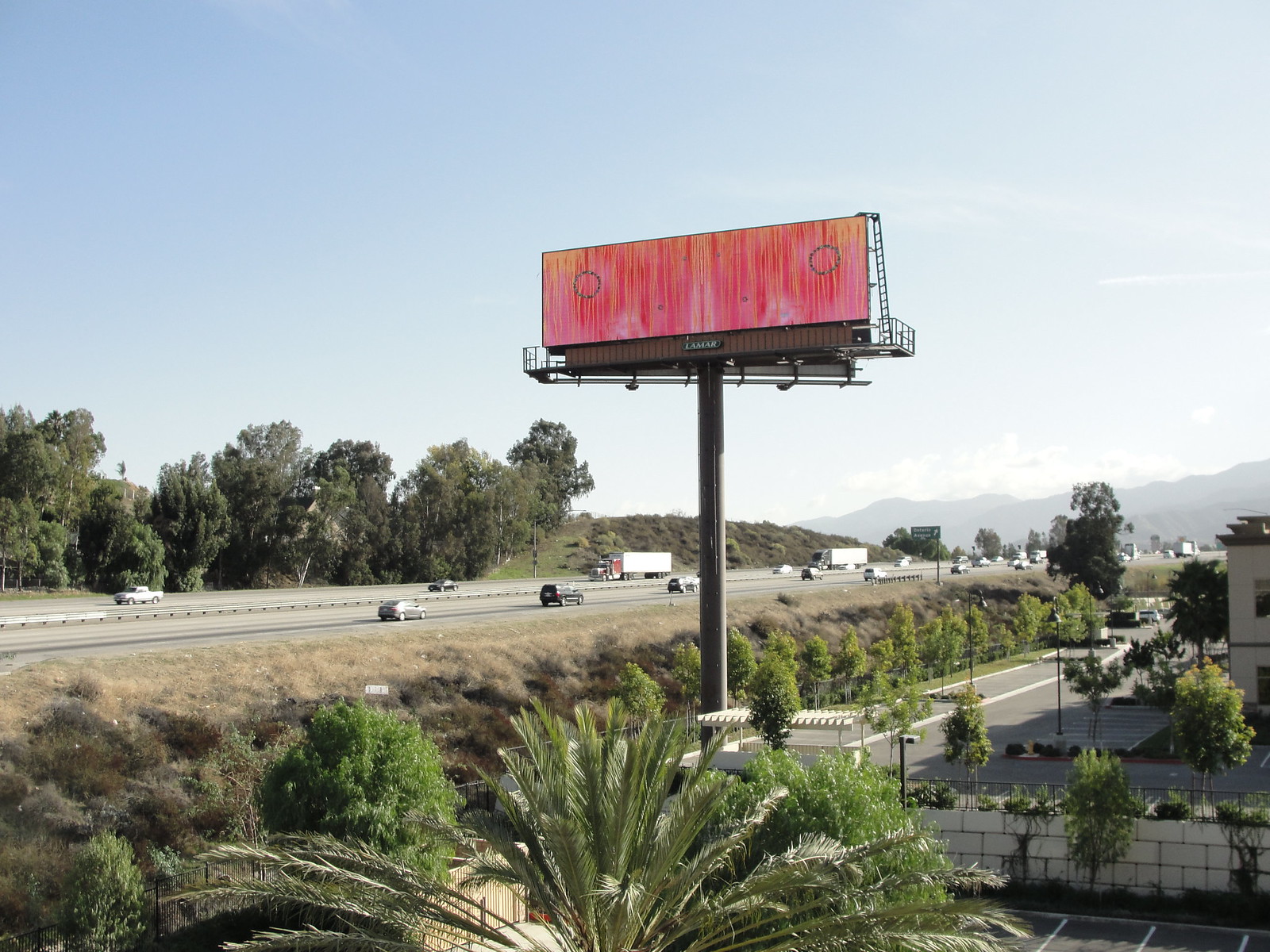This outdoor photograph captures a scenic view of an interstate highway running horizontally across the image, with visible traffic including cars, sedans, trucks, and large tractors traveling in both directions. The highway is bordered by green trees and foliage on the far side, with a prominent hill rising behind them. In the foreground, there are sloped embankments leading down to a parking lot protected by a giant concrete wall. This lot features white parking lines and is home to a building located on the right side of the image. In addition, several palm trees stand directly in front of the camera. Centered in the scene is a large metal billboard with a red and orange background; the upper part of the billboard includes a green section with white text saying "Lamar," while a brown background occupies the lower section. The sky above is a gradient of light to darker blue with partial cloud cover. In the distant background, a picturesque mountain range completes the landscape.